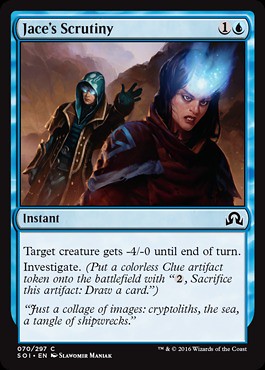This image features a detailed scan of a fantasy trading card titled "Jace's Scrutiny." The card's layout includes a black outer border with a smaller blue border inside it. At the top of the card, within a light blue oval area, the title "Jace's Scrutiny" is displayed prominently. The central illustration depicts a stern-looking woman with mystical light radiating from her forehead, casting bright stars. She appears menacing, dressed in a fantasy outfit with a cloak. Behind her stands a young man in a hoodie and glasses, his open palm raised behind her head, emitting the same mystical light from his eyes. They are set against a backdrop of dark brown smoke clouds. The area below the illustration contains the word "INSTANT" in black text. Further down, in a white rectangle, is the text: "Target creature gets -4/-0 until end of turn. Investigate. Put a colorless Clue artifact token onto the battlefield with, 'To sacrifice this artifact, draw a card.'" The card blends a collage of images, including phrases like "Cryptolith's the sea, a tangle of shipwrecks," adding to its mysterious and intricate design.